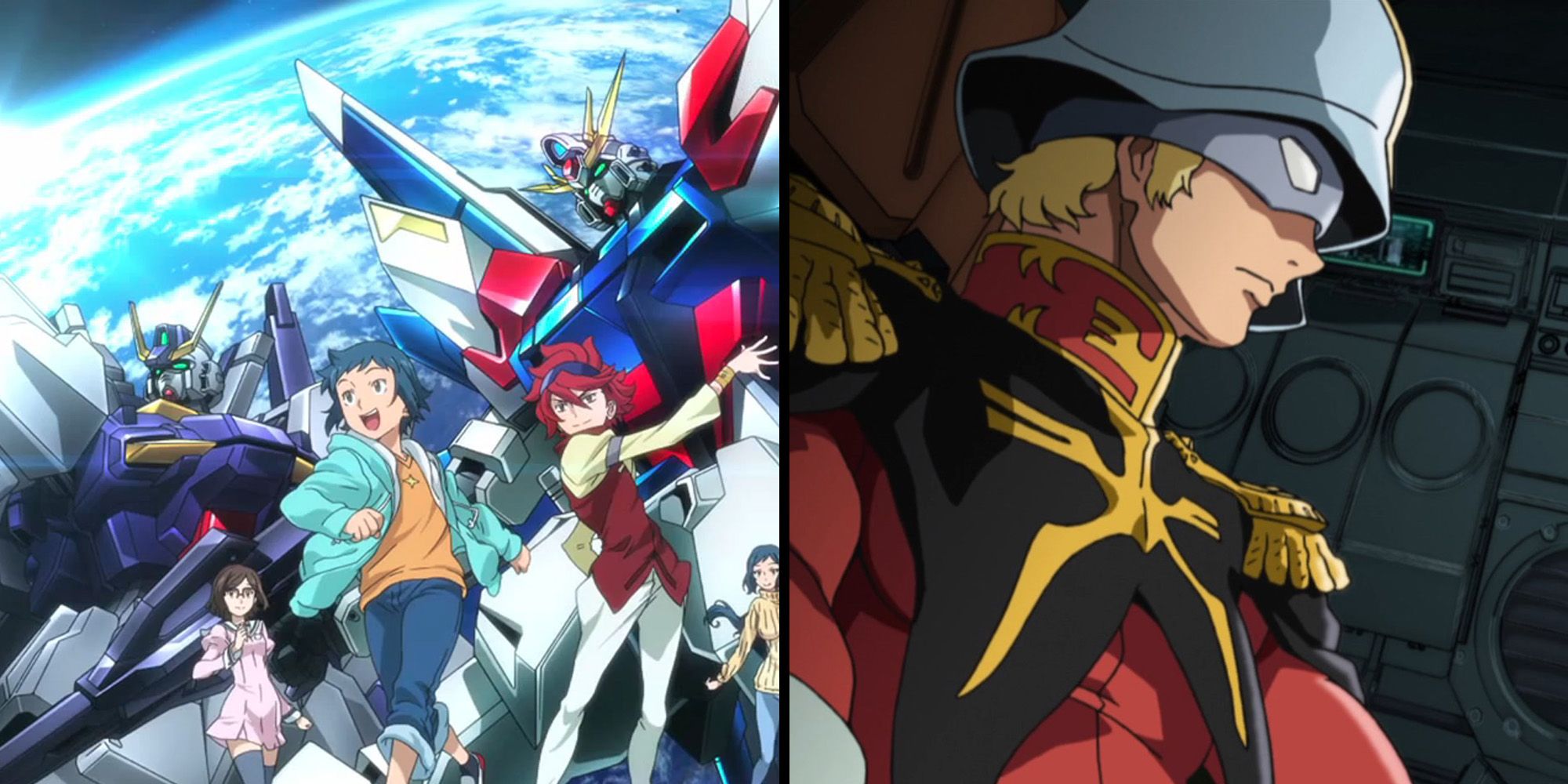This anime cartoon image is divided into two parts. On the left side, there's a planetary backdrop with the Earth visible above. In the sky, two towering mecha robots in white, blue, and red colors dominate the scene. Below them, various characters stand out. A young kid with spiky black hair and blue, cuffed jeans is at the center, donned in a blue jacket and an orange shirt. To the left, a girl in a pink dress and glasses, wearing stockings, stands near another character whose outfit includes a red vest and white pants. Further right is a woman in a white sweater, partially visible in the background. On the right side of the image, there's a military-like figure inside what seems to be a spaceship. This character sports a black naval uniform with gold tassels on the shoulders and a red shirt underneath. He wears a silver helmet with a visor, hinting at a commanding or captain role.